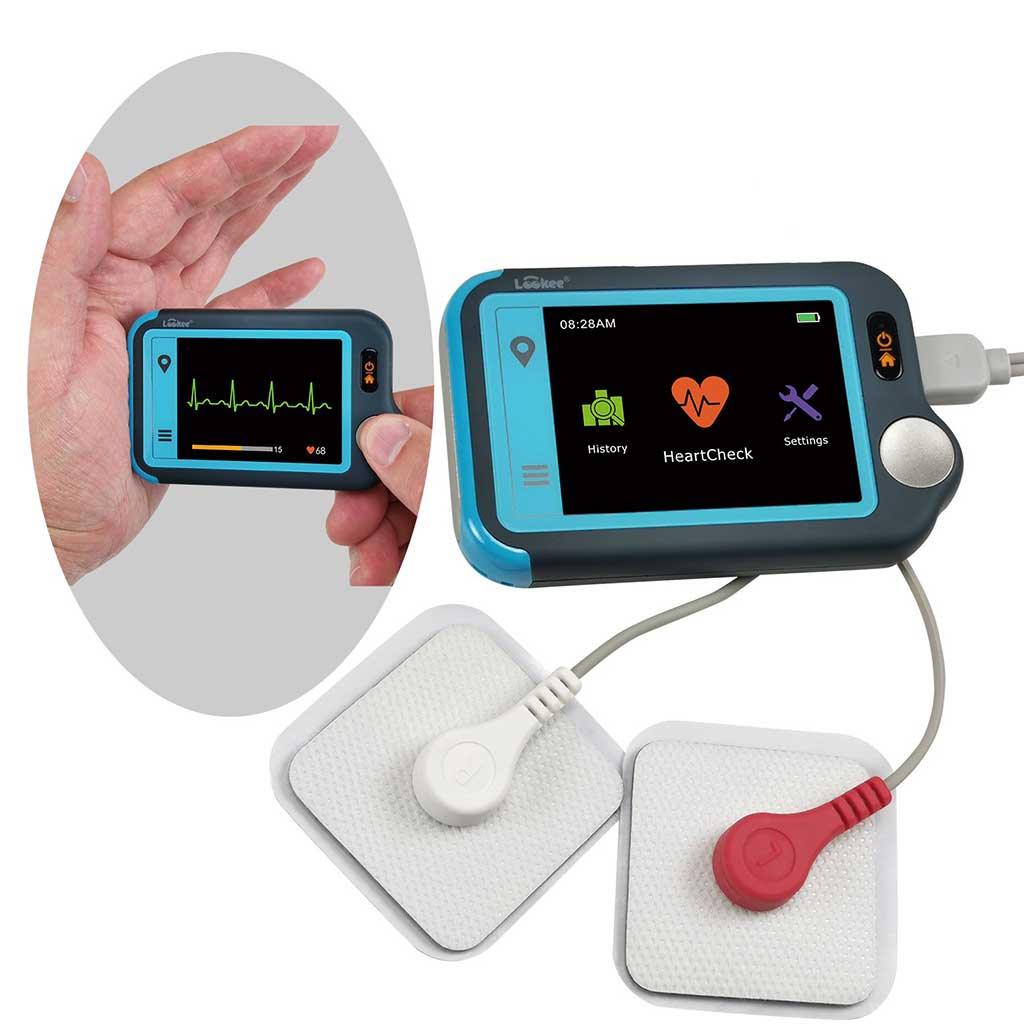This image features a close-up, advertisement-style photograph of a heart rate monitor against a completely white background. Dominating the left side is an oval inset depicting a person's left palm open wide, with the person pressing the device into their palm, suggesting it may be recording heartbeats or blood pressure. The heart monitor itself is a rectangular device in shades of gray and blue with a black screen displaying various functionalities. The top left of the device features the brand name "Lookee." 

On the monitor's screen, there are labels: "Heart Check" with an orange symbol of a red heart encompassing an EKG line, "History" with a green magnifying lens icon, and "Settings" with a purple icon of a screwdriver and wrench. A yellow bar and green pulse waves mimic those seen on medical equipment, indicating live heart rate data. The device also shows a small battery logo and time. Notably, it has two wires—one gray and one red—each attaching to patches meant to be applied to the user's skin.

The main colors in the image include black, white, different shades of gray, pink, green, yellow, blue, red, purple, and orange. The detailed depiction and color coding make it clear that this health monitor offers various features for tracking cardiac health, including history monitoring and settings adjustments.